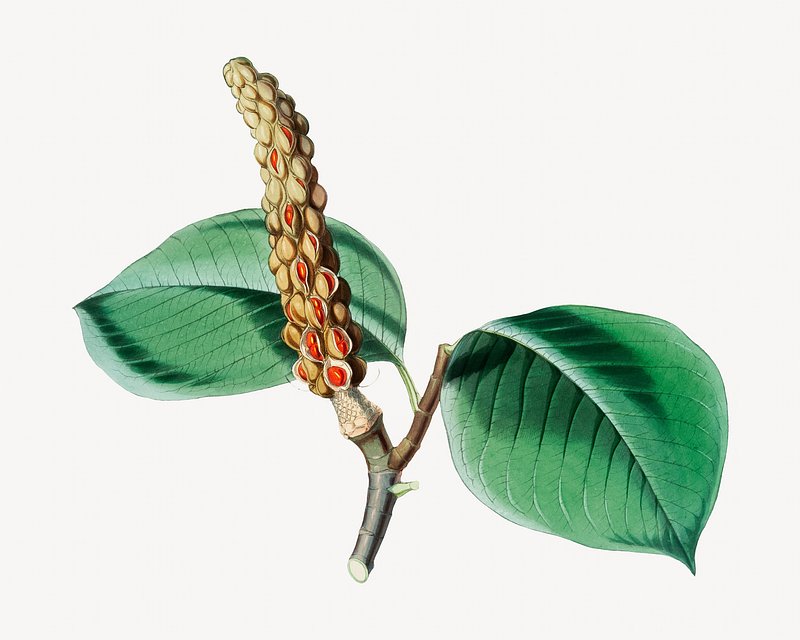This image showcases a detailed illustration of an unidentified plant against a completely white background. Central to the composition is a grayish main stalk from which a brown secondary stalk branches off. This secondary stalk supports two large, dark green leaves with visible veining, shining as if bathed in light. Above the leaves, emanating from the main stalk, is a prominent, column-like structure covered in numerous tan seed pods. These pods are in various stages of opening, revealing vibrant red seeds within. The bottom part of this structure, where the branch appears cut off, accentuates the natural texture and intricacy of the plant’s design. The overall effect is both striking and meticulous, bringing attention to the plant’s complex and rich details.